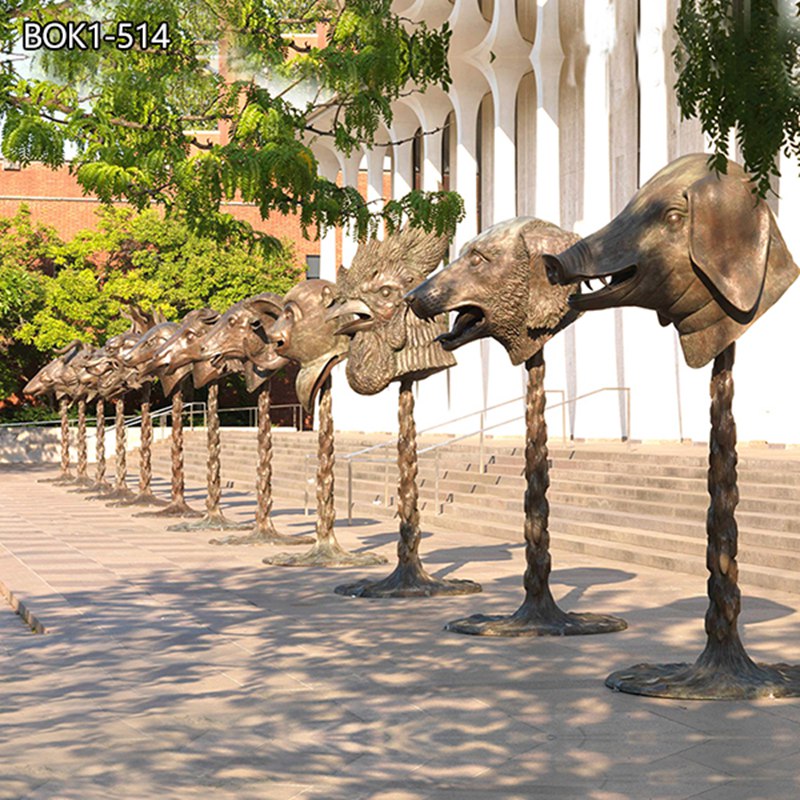The image depicts a white building with tall columns and a series of steps leading up to it, situated in the right upper corner. Metal banisters flank the steps, which descend to a stone tile ground. In front of the building, there is a row of approximately a dozen animal head statues on twisted, braided poles. These statues appear to be sculpted from a reddish-gray material, possibly stone or metal. Among the identifiable animal heads are a monkey, rooster, dog, wild boar, goat, and horse. Overhead, yellowish-green leaves from nearby trees partially cover the scene. There is also text in the top left corner that reads "BOK 1-514." Shadows cast by the surrounding elements add depth to the image.